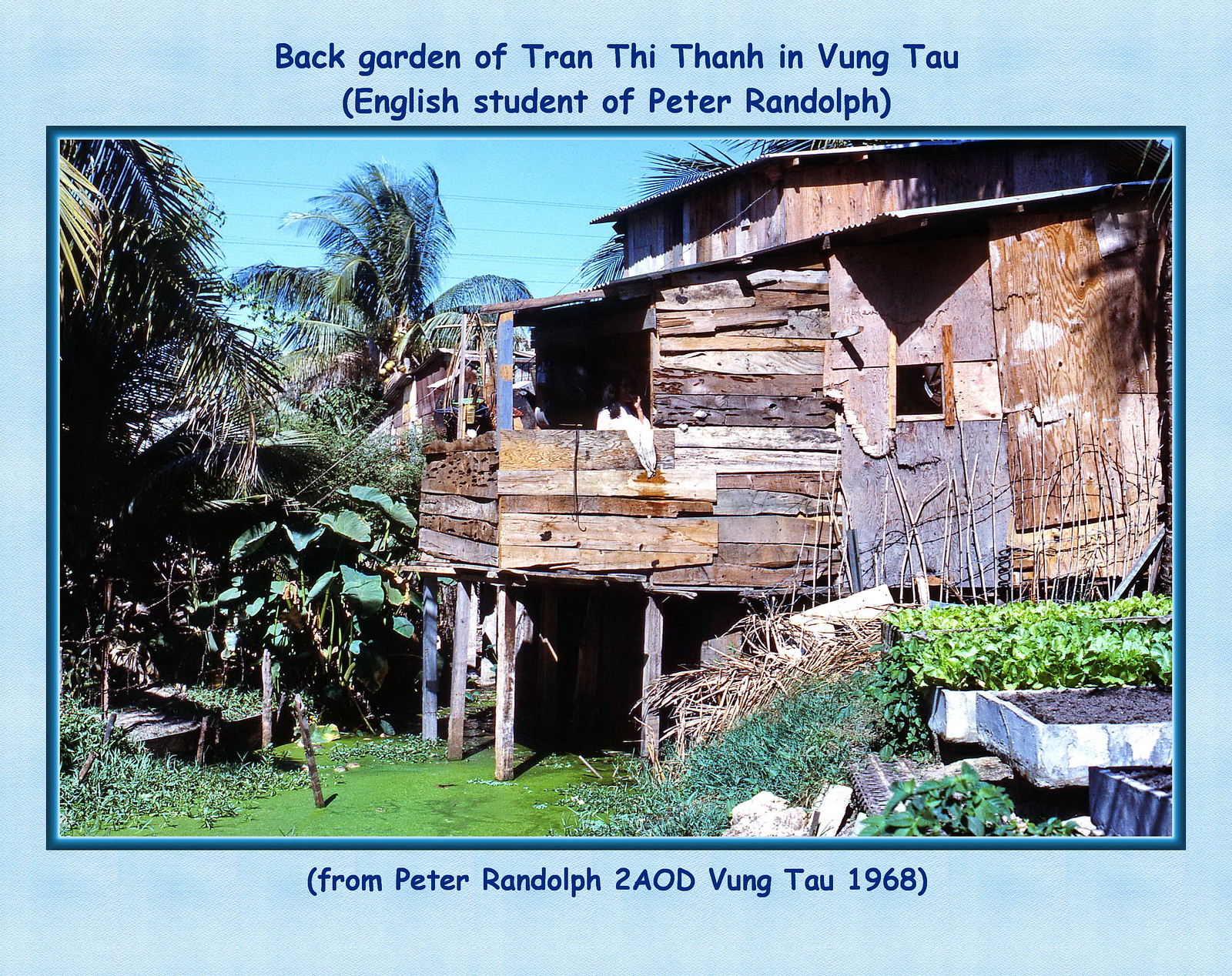The image depicts a ramshackle wooden structure that appears to be hastily assembled from variously colored planks, ranging from very light to dark brown hues. This haphazard building is partially elevated on stilts on its left side, creating an open space underneath, while its right side rests directly on the ground. The area below the stilts is covered in bright green, which could either be grass or still water, giving it a swamp-like appearance. Surrounding the structure is a lush environment with tall green palm trees and other greenery, set against a backdrop of clear blue sky with visible power lines. The building itself lacks proper windows; instead, there are small or non-existent openings where wood is absent. A person, likely a woman, can be faintly seen inside, facing away from the camera.

The photograph is bordered by a light blue frame with dark blue text. At the top of the image, the caption reads, "Back Garden of Tran Thi Thanh in Vung Tau," with "English student of Peter Randolph" noted in parentheses. Below the picture, another inscription in parentheses states, "From Peter Randolph to AOD, Vung Tau, 1968." The scene captured in the photograph evokes a sense of fragility and improvisation, typical of shelters found in underdeveloped regions.